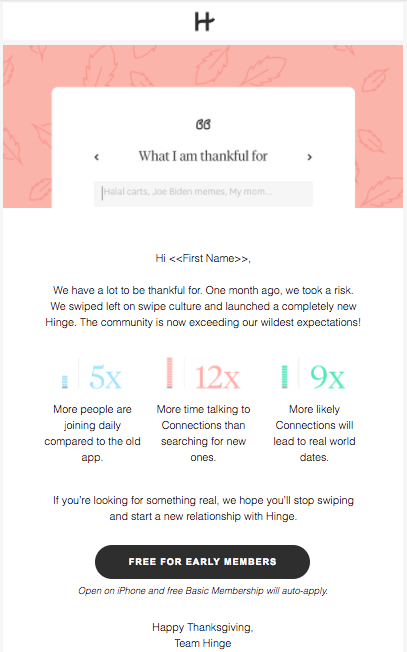A screenshot of a website features a cohesive and visually appealing layout. At the top, a white banner prominently displays a black cursive 'H,' signifying the Hinge logo. Below the banner, a salmon-pink section is adorned with delicate pink leaf icons. Within this area, a white box contains text reading "What I'm thankful for," accompanied by what appears to be a '66' at the top, though it might be stylized quotation marks.

Further down, there's a search box with options such as 'cards,' 'Joe Biden memes,' and 'my mom.' Following this, black text greets the user with "Hi, [first name], we have a lot to be thankful for. One month ago, we took a risk. We swiped left on Swipe Culture and launched a completely new hinge. The community is now exceeding our wildest expectations."

Continuing downward, the text highlights key achievements: in blue '5X' with a blue icon indicating more daily users compared to the old app; in salmon-pink '12X' with a pink icon showing increased conversation time with connections versus searching for new ones; and in green '9X' with a green icon reflecting a higher likelihood of real-world dates.

The section concludes with an invitation in black text to stop swiping and start meaningful relationships with Hinge. A black box further emphasizes that the app is free for early members, with instructions to 'Open on iPhone' and an assurance that the basic membership is automatically applied. The message ends with a holiday greeting: "Happy Thanksgiving, Team Hinge."